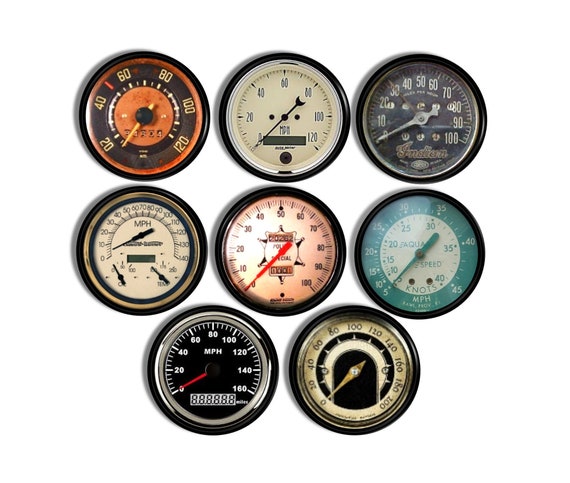The image showcases eight vintage speedometers arranged in three rows against a neutral background. The top row consists of three speedometers: the leftmost speedometer features an orange center with an orange outer ring, white numbers ranging from 20 to 120, and black markings; the middle speedometer is predominantly white, featuring both analog and digital elements, and ranges from 0 to 120; the rightmost speedometer has a dark gray face with white numbers and markers, ranging from 0 to 100. The middle row also contains three speedometers: the leftmost is black and white with numbers for miles per hour and also shows smaller, less discernible gauges; the central speedometer is unique with a reddish tint and a red dial, likely incorporating elements beyond just speed; the rightmost is dark teal with white fonts. The bottom row has two speedometers: the leftmost is black with a digital counting feature at the bottom; the rightmost is black with gold accents. All the dial hands are uniformly pointing to the bottom left, and these speedometers reflect a variety of styles and eras, with some capable of reading in miles per hour and others in kilometers.